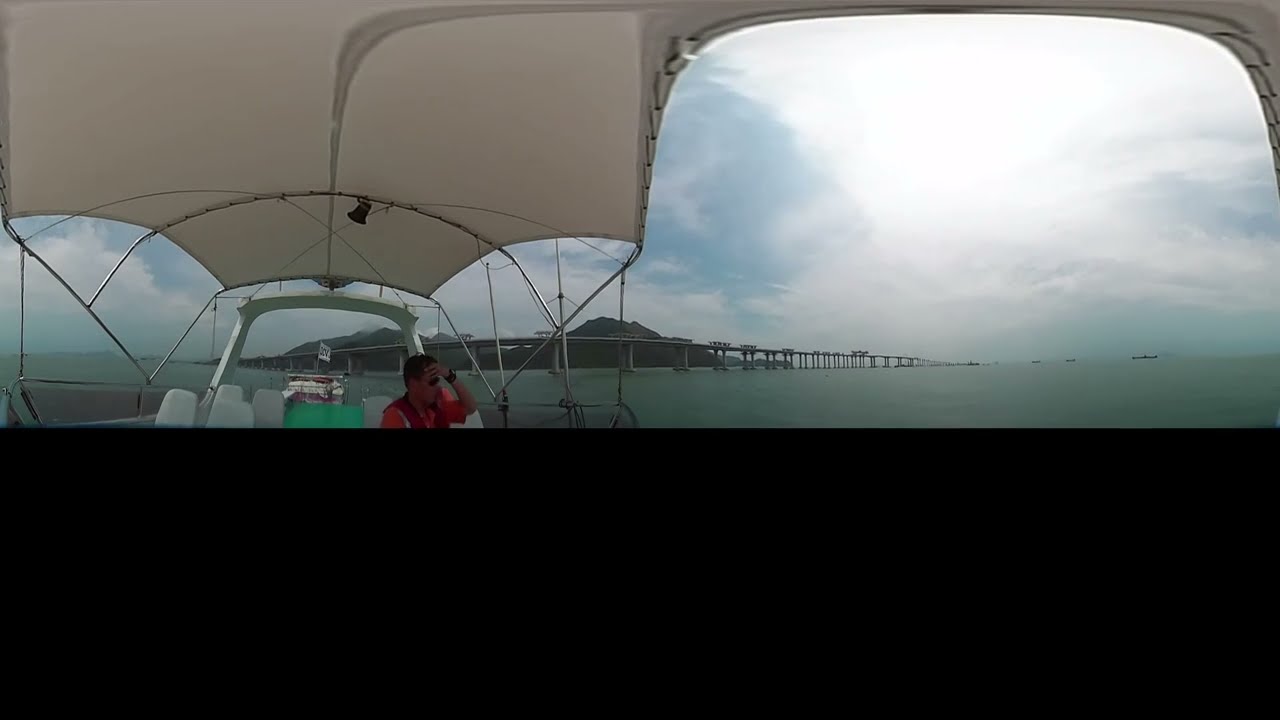The image captures an outdoor scene from the perspective of inside a boat navigating a green-tinted waterway. The boat, featuring white seating and a canopy held up by metal scaffolding, has a person with dark hair wearing a red shirt and glasses. This individual is seated and looking towards the right. The waterway is spanned by a bridge that stretches from the left across the horizon, coming closer to the foreground, and then fading away into the distance. The sky above is partially cloudy, allowing some light to filter through, indicating a daytime setting. In the backdrop, a small hill or mountain adds to the landscape. The bottom section of the image appears blacked out or cut off, but it does not detract from the detailed view of the person on the boat amidst this serene, multi-layered scenery.